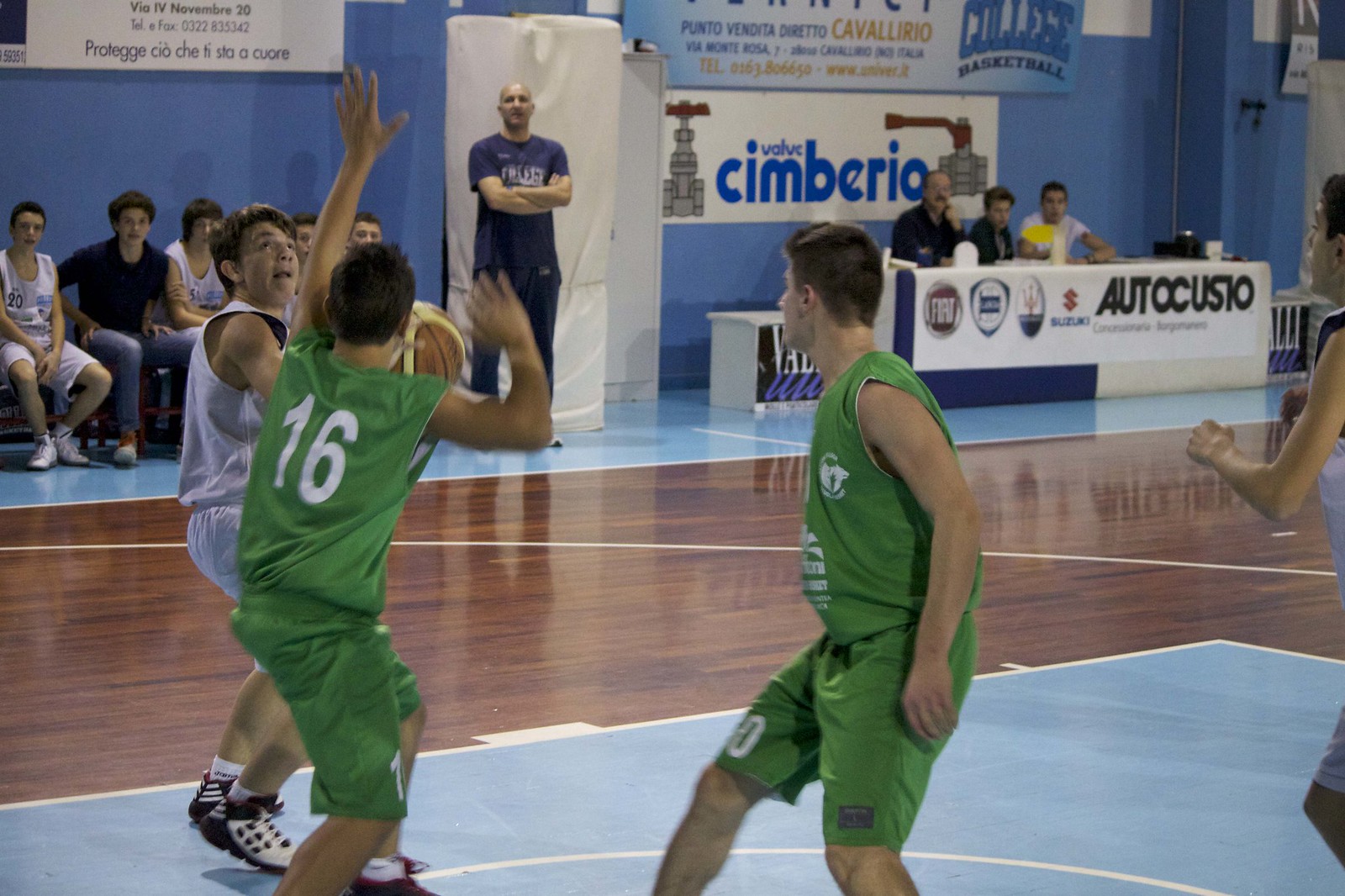The image depicts a high school basketball game in progress, set in a well-lit interior gymnasium with a polished wooden floor featuring blue-painted areas marking the shooting zone. The focus is on a tense moment where a player in a green jersey and shorts, numbered 16, raises his arms to block an opponent. This opponent, dressed in a blue jersey and white shorts, holds the basketball with a determined expression, seemingly preparing to take a shot. Surrounding them are additional players in similar green and blue attire. On the sidelines, a group of teenagers can be seen, some seated and others standing, while a man dressed in a blue shirt and jeans watches attentively, possibly a coach. Behind them is a table with three adults, possibly officials or scorekeepers, beneath banners and advertisements that include the names "AutoCuzio" and "Values, Simbirio," some of which are in a foreign language. Despite only capturing a portion of the court, the image vividly conveys the competitive and immersive atmosphere of the ongoing game.